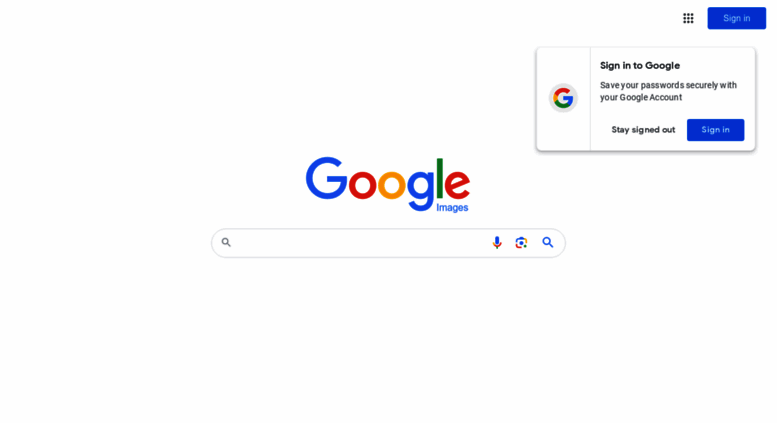The image depicts the homepage of Google Images with a clean, minimalist design dominated by a stark white background. Centrally positioned is the iconic Google search bar, prominently labeled "Google Images." The word "Google" is displayed in the company's bold, signature font, with the letters colored in the standard Google palette: blue for the "G," red for the first "O," yellow for the second "O," blue for the second "G," green for the "L," and red for the "E." 

In the upper right-hand corner, a "Sign in" button is visible, accompanied by a pop-out tooltip that prompts users to sign into their Google account for enhanced security features, offering options to stay signed out or to sign in. The tooltip also features the colorful Google "G" logo. 

Within the search bar itself, aligned to the right, there is a microphone icon, indicative of voice search functionality, followed by an image icon to facilitate searches by image, and finally the standard magnifying glass icon, denoting the search action.